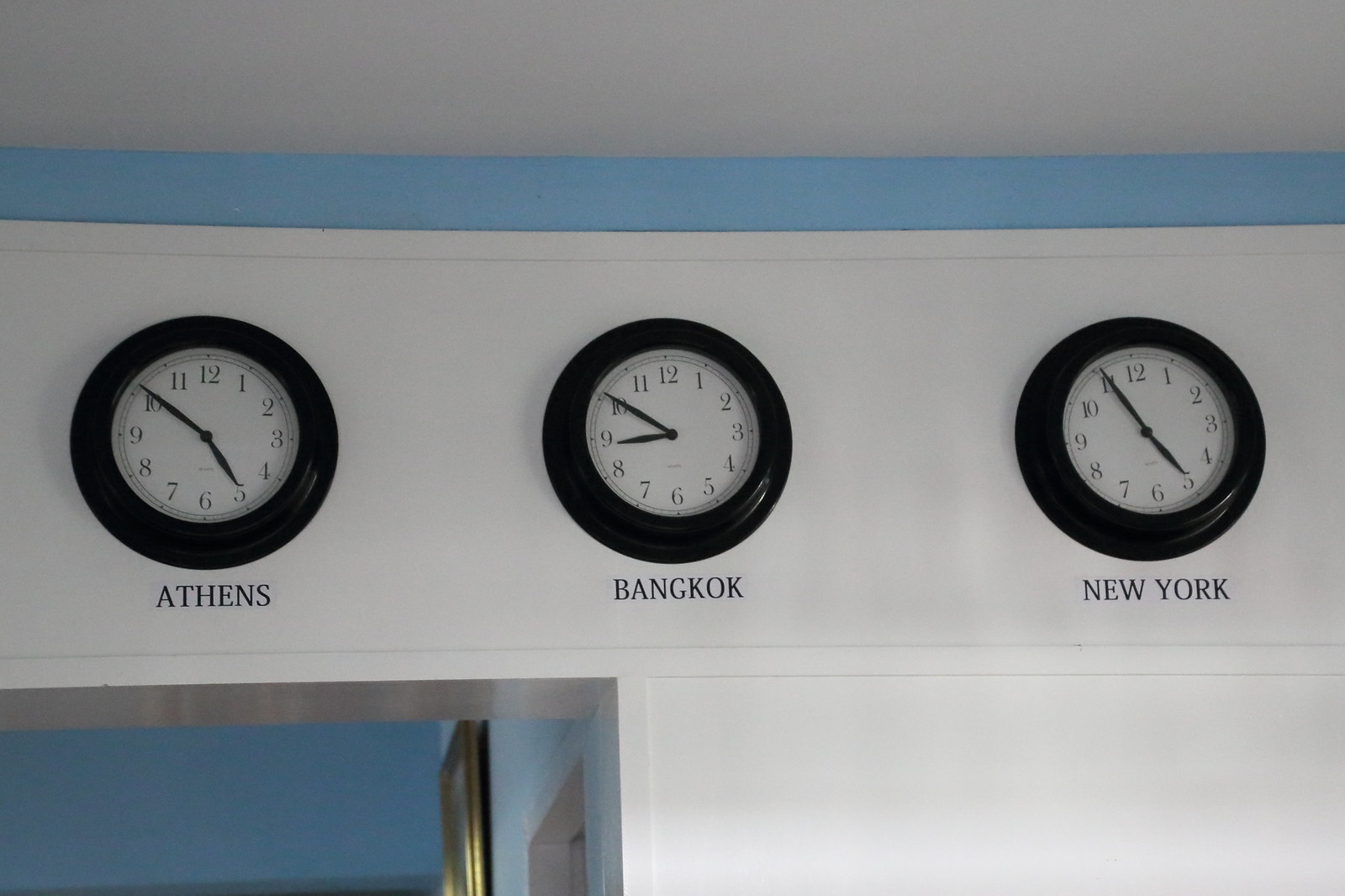In this landscape-oriented photograph taken indoors, the upper part of a white wall is adorned with three identically rimmed black clocks, each with a white face featuring black numbers, hour hands, and minute hands. Near the ceiling, the wall transitions to a pale blue shade. From left to right, the first clock with “Athens” in black font underneath displays a time of 5:51. The middle clock, labeled “Bangkok,” shows the time as 8:51. The final clock, marked “New York,” reads 4:55. The image also captures part of a doorway with an open door, revealing a glimpse into another room where a gold-framed picture can be seen on the wall, and part of the ceiling in that room is visible.